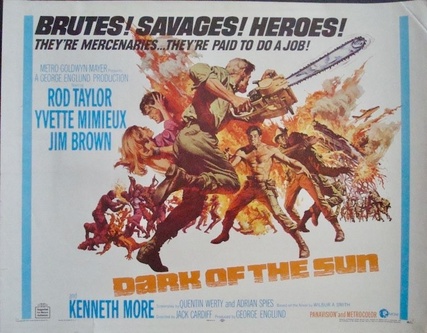The image is a color photograph of a vintage movie poster, likely from the late 1960s. Dominating the top, bold black letters declare "BRUTES, SAVAGES, HEROES." Underneath, in smaller type, the poster clarifies "They're mercenaries. They're paid to do a job." The central image features a dramatic scene: a man clad in army clothes brandishes a chainsaw, seemingly lunging toward a shirtless man, set against a backdrop of explosive action. Surrounding the central conflict are various action scenes, including a man and woman on the verge of kissing. Below, in prominent orange letters, the title "Dark of the Sun" is displayed. Actor names appear in blue font to the side: Rod Taylor, Yvette Mimieux, and Jim Brown. The backdrop is a clean white, enhancing the retro action vibe of the poster.